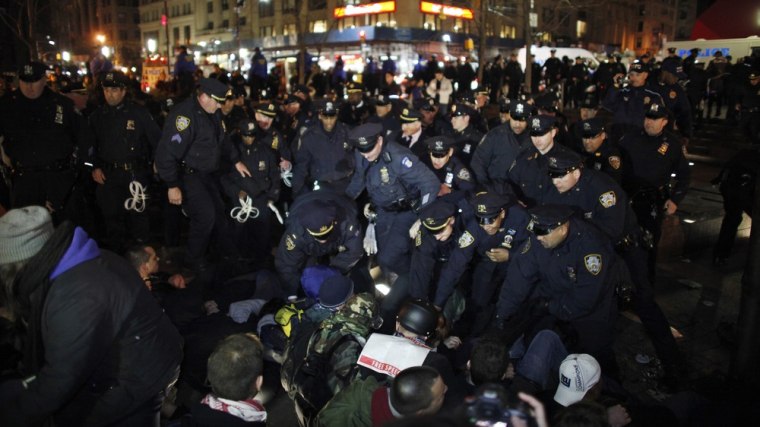This nighttime city photograph captures a tense scene with a considerable number of police officers lining up, clad in dark blue uniforms, including button-down shirts, matching pants, hats, and some in jackets, suggesting chilly weather. The officers in the front row appear to be linking arms, with a few reaching down towards a group of individuals sitting on the ground in front of them, potentially engaged in a sit-down protest. These individuals, likely men, are dressed in coats and some are wearing hats or toboggan caps. Behind the officers, the city's tall concrete buildings and lights frame the backdrop, while the situation’s atmosphere is somewhat ambiguous, as the officers do not seem aggressively engaged despite the protest-like setting.